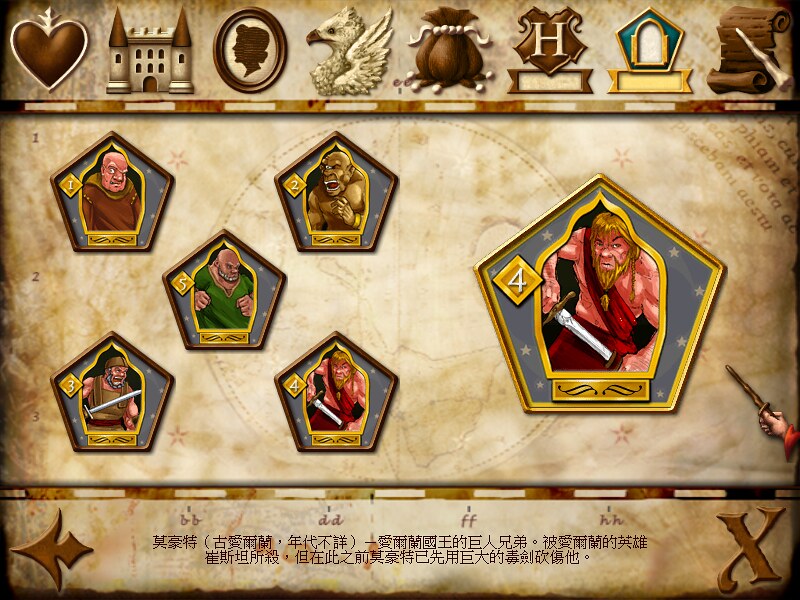The image appears to be a digitally created, top-down view of a board game or a still from a video game, primarily set on a beige background resembling a map. The center of the image features a circular world map, while the border at the top and bottom is accented with brown and beige. At the top, there is a decorative banner featuring various brown and beige icons including a castle, a silhouette of a woman's face, an eagle, a decorative bag, the letter 'H', and a scroll with a writing tool.

Below the banner, six numbered hexagonal or pentagonal shapes each contain different character illustrations that seem to be from a medieval or fantasy setting. These characters, resembling superheroes or warriors, include a man with red skin and a yellow beard wielding a sword, another man with a sword, an ogre-like figure with an open mouth, a caveman, and a bald man in a fighting stance wearing a brown outfit. Along the bottom edge of the image, there are some Asian or Chinese calligraphy symbols and an 'X' to the right of the text.